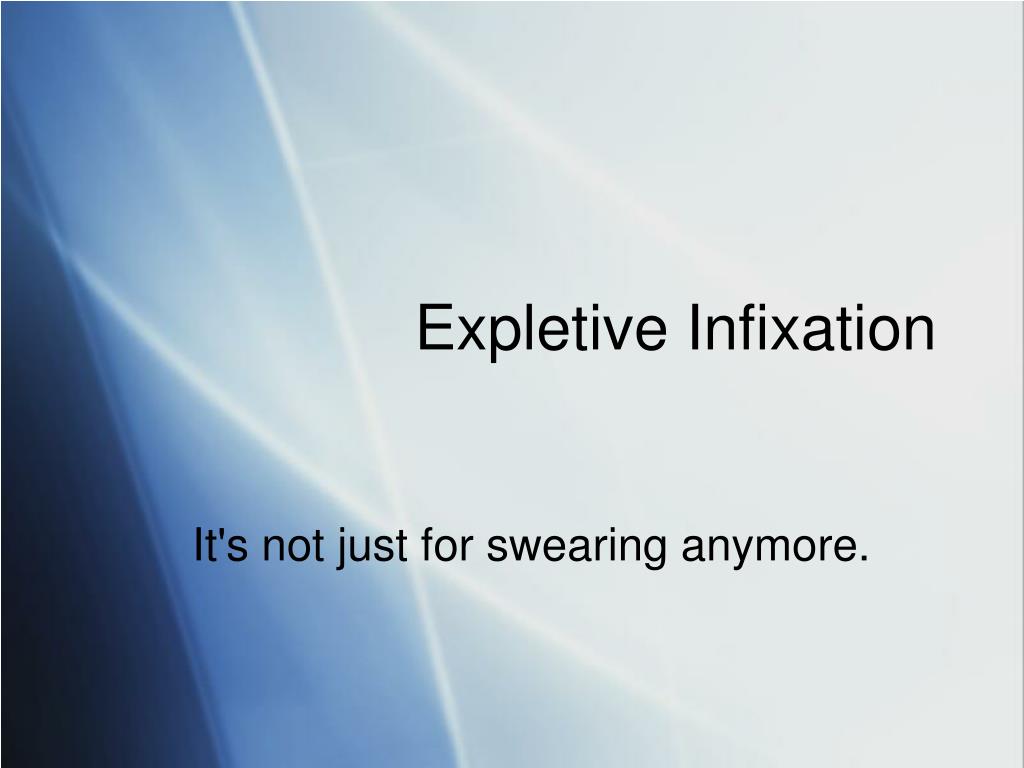The image is a PowerPoint slide featuring bold, black text centrally aligned on a stylized geometric background. The text at the center reads "expletive in fixation" in large letters, with a smaller line below stating, "It's not just for swearing anymore." The background primarily consists of light blue, with two vertical stripes on the left edge transitioning from navy blue to powder blue as they extend from the bottom to the top of the slide. Additionally, diagonal sections on the left subtly shift in shades from light to dark blue, adding a dynamic visual element to the backdrop.